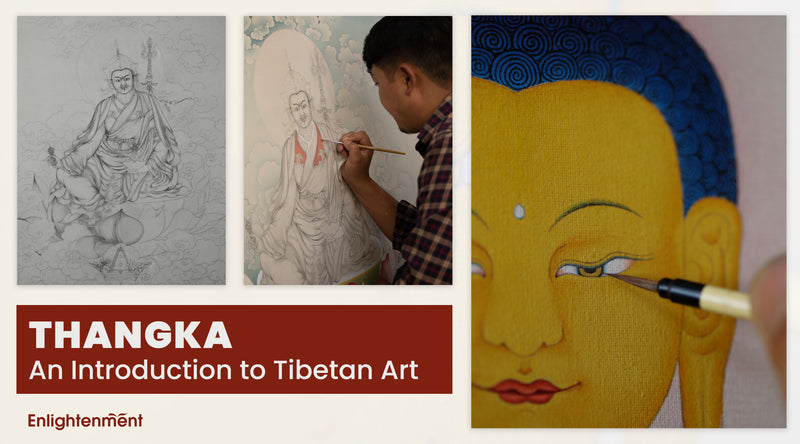This image appears to be an advertisement or flyer for learning Thangka, a traditional Tibetan art form. Set against a white or off-white background with a white border around each section, the layout includes three key images. On the left, two smaller images are stacked vertically. The top one depicts an initial pencil drawing of a robed figure, possibly holding a weapon like a sword or spear and wearing a helmet. Below this, a man in a checkered shirt is seen adding an orange hue to the same drawing with a paintbrush. To the right, a larger close-up image showcases the intricate detail of the art, focusing on the head of the figure, with yellow skin and blue, swirling hair, and a hand meticulously painting the eye with a yellow shade. Positioned beneath the two left images is a red banner with the text "Thangka, an introduction to Tibetan art," and "Enlightenment" written below it in red font, emphasizing the theme of exploring Tibetan artistic and spiritual heritage.